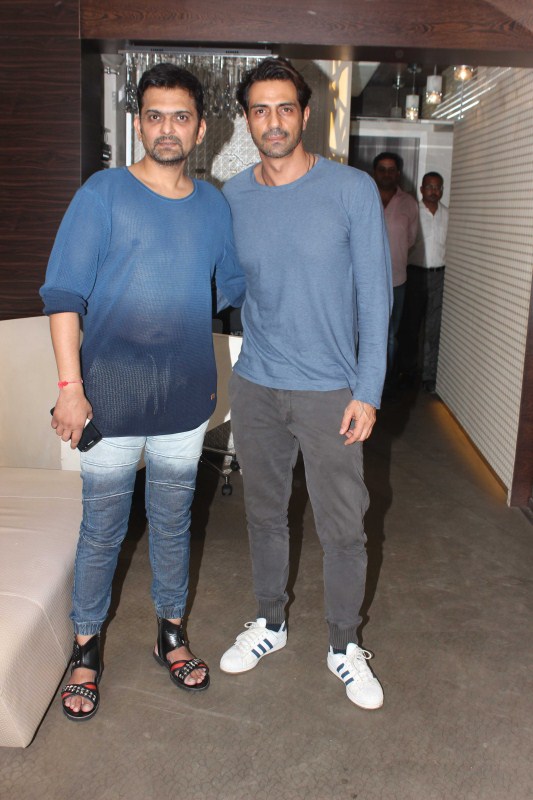In this indoor color photograph, two middle-aged men, likely in their late 30s, are standing side by side and looking up at the viewer, smiling. They both have dark hair and scruffy beards. The man on the left is wearing a blue mesh long-sleeved shirt with the sleeves rolled up, faded blue jeans, and black sandals. The man on the right is dressed in a long-sleeved light blue shirt, dark gray pants, and white sneakers. They have their arms around each other, suggesting camaraderie. 

The setting includes a room with dark wooden archways and walls, and a partially visible white wall with gray lines running across it on the right-hand side. Behind the two men, there is a white couch to the left and a silver or white wall that's difficult to discern in detail. The floor appears gray. In the far background, two more men, one in a pink shirt and the other in a white shirt, can be seen standing distantly. This photograph is in portrait orientation and is a part of a Bollywood meetup event, featuring actor Arjun Rampal joining the cast of "Ankhon 2."